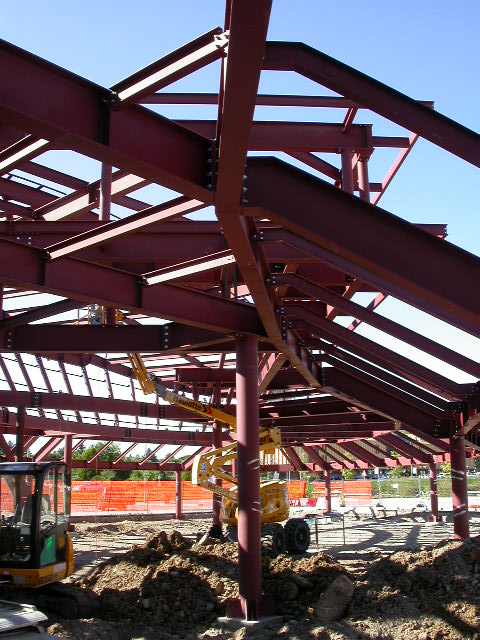The image depicts a bustling construction site dominated by a large, rusty reddish metal structure that appears chaotic and twisted, possibly in the process of being either constructed or dismantled. At the forefront, a yellow cherry picker is elevated to the top of this metal framework, its bright color contrasting with the dark, rusty beams. Nearby, a small backhoe is positioned underneath the metal structure, indicating active site work. Towards the front, a mound of freshly dug dirt highlights ongoing excavation efforts. The background features an orange mesh fence demarcating the construction area from a parking lot, with hints of grass and trees visible farther back. The scene is set on a sunny day, adding a stark clarity to the construction activities and surroundings.